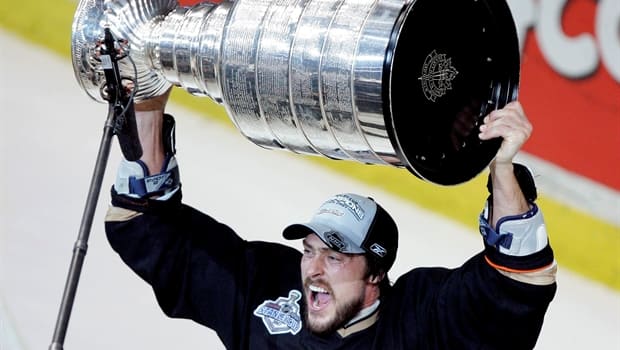In the image, a jubilant hockey player is holding up a sizeable silver trophy, likely the Stanley Cup, in a sideways position, with his left hand on the top and his right hand on the bottom. He is visibly ecstatic, with his mouth wide open in a triumphant scream, showcasing his teeth. He is dressed in a black jersey, displaying what appears to be the partially visible word "Stan" and a badge, though specifics are grainy. His attire includes a very dark blue, long-sleeve jacket, suggesting a hockey ensemble, and he sports a short brown beard. His head is covered with a gray and black baseball cap, prominently featuring the word "Champions" and a logo on the left side of the black section at the back of the cap. The background suggests the setting might be an ice rink, with a blurred white surface underfoot and a red wall with white and yellow stripes behind him. A microphone juts into the frame from the bottom left corner, aimed toward him and the trophy, adding to the celebratory atmosphere. Only the upper part of his body is visible, emphasizing his emotional victory moment.